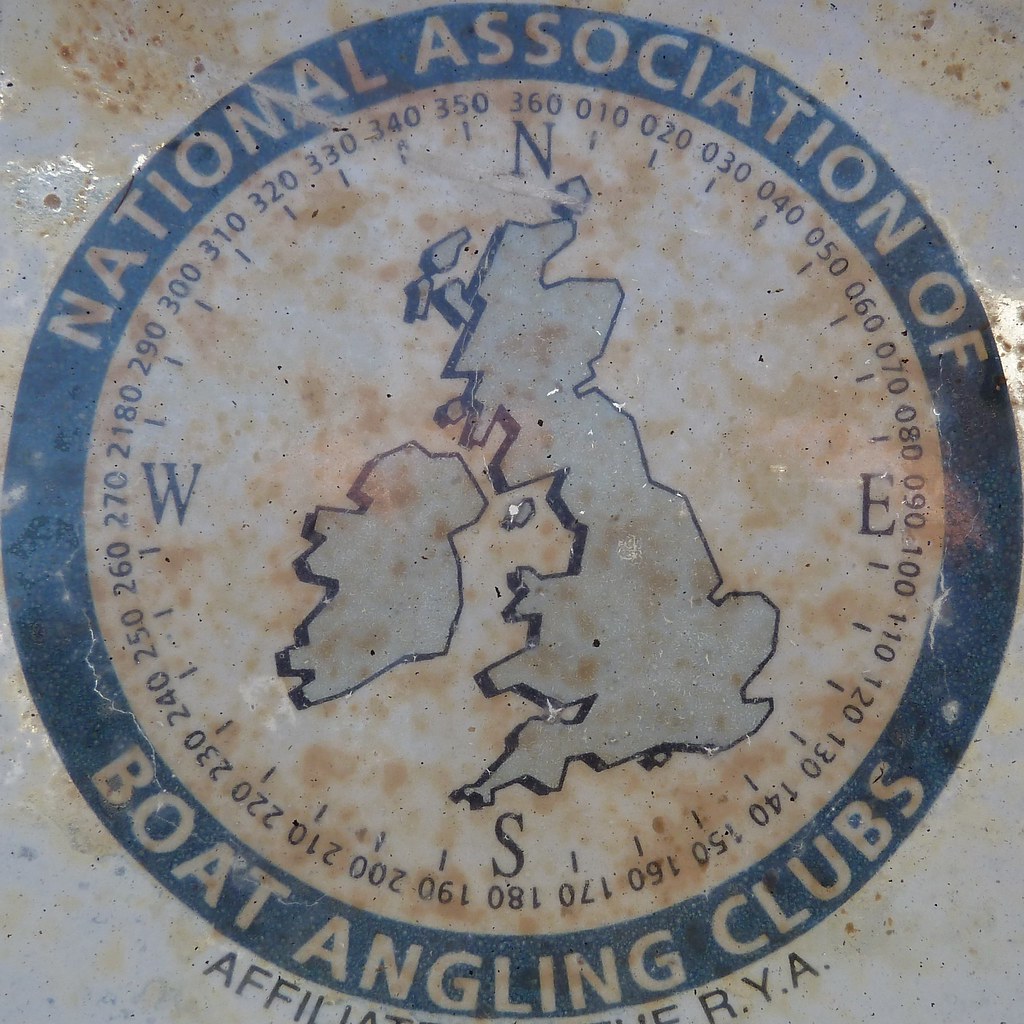This close-up color photograph captures a weathered logo painted on the side of a rusted metal surface, possibly a boat. The background is a dirty, whitish-blue with rusty brown patches, indicating exposure to water and elements. The circular logo is prominently centered and encircled in blue, with the words "National Association of Boat Angling Clubs" around the edge. Inside the blue border, the logo features a compass design with cardinal directions marked by N, E, S, and W, and numerical compass points graduating by tens, from 360° at North to 180° at South. The core of the logo features a blue and white map of the UK, further emphasizing its nautical theme. The entire scene appears grimy, with smudges and potential remnants of spilled liquid adding to its rugged seafaring character.